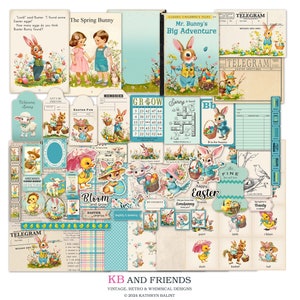The image features a collection of vintage Easter-themed children's stories and Easter cards, rich in nostalgic illustrations and vibrant colors like yellow, pink, and blue. The centerpiece is a storybook titled "Mr. Bunny's Big Adventure," showcasing a bunny dressed in a vest and suit. Surrounding the book are various pieces of Easter paraphernalia, including stickers of cute little bunnies, small yellow ducks, and a little bluebird sticker prominently in the center. Visible text includes cheerful phrases like "Happy Easter," and there are postcards depicting children holding hands. Some pages from the book are adorned with colorful illustrations and short paragraphs, indicating it's tailored for young readers. The narrative appears playful and whimsical, featuring human-like animals, including a bunny walking on two legs and engaging in activities like collecting Easter eggs with two young children. A small telegram of a bunny is seen at the bottom left, and a notable label reading "KB and Friends" is present at the very bottom. Other text remains largely illegible.